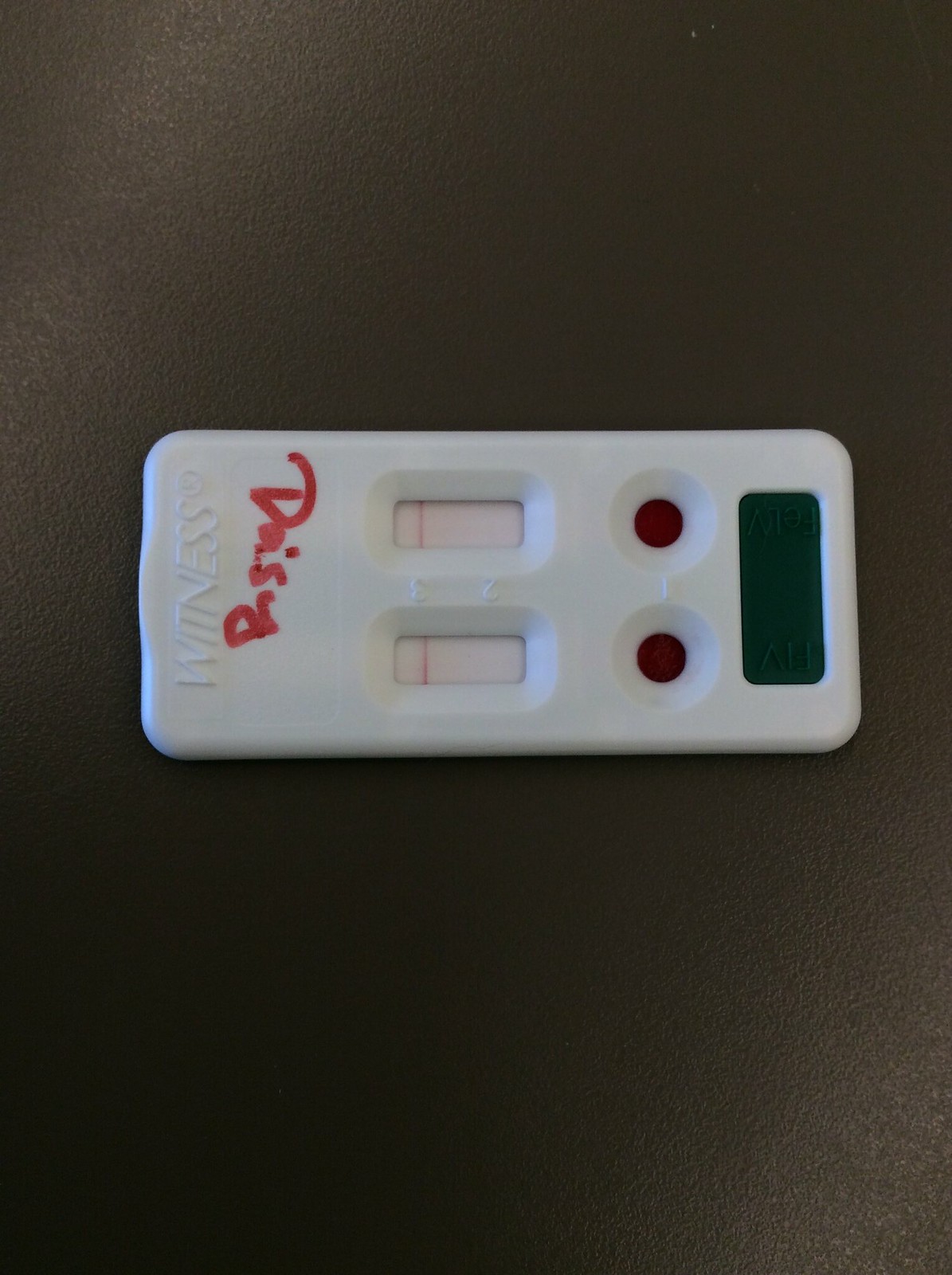In this image, a white plastic component resembling a pregnancy test is placed on a black tabletop. The device features two embedded red circles aligned vertically. Above these circles is a dark green rectangle. Additionally, there are two indents on the component, each containing a solid line. The name "Wenness" is displayed prominently on the device. Written in red marker, there appears to be a name, although it is difficult to decipher. The component also has the numbers "2" and "3" engraved on the plastic surface, adding to its detailed design.